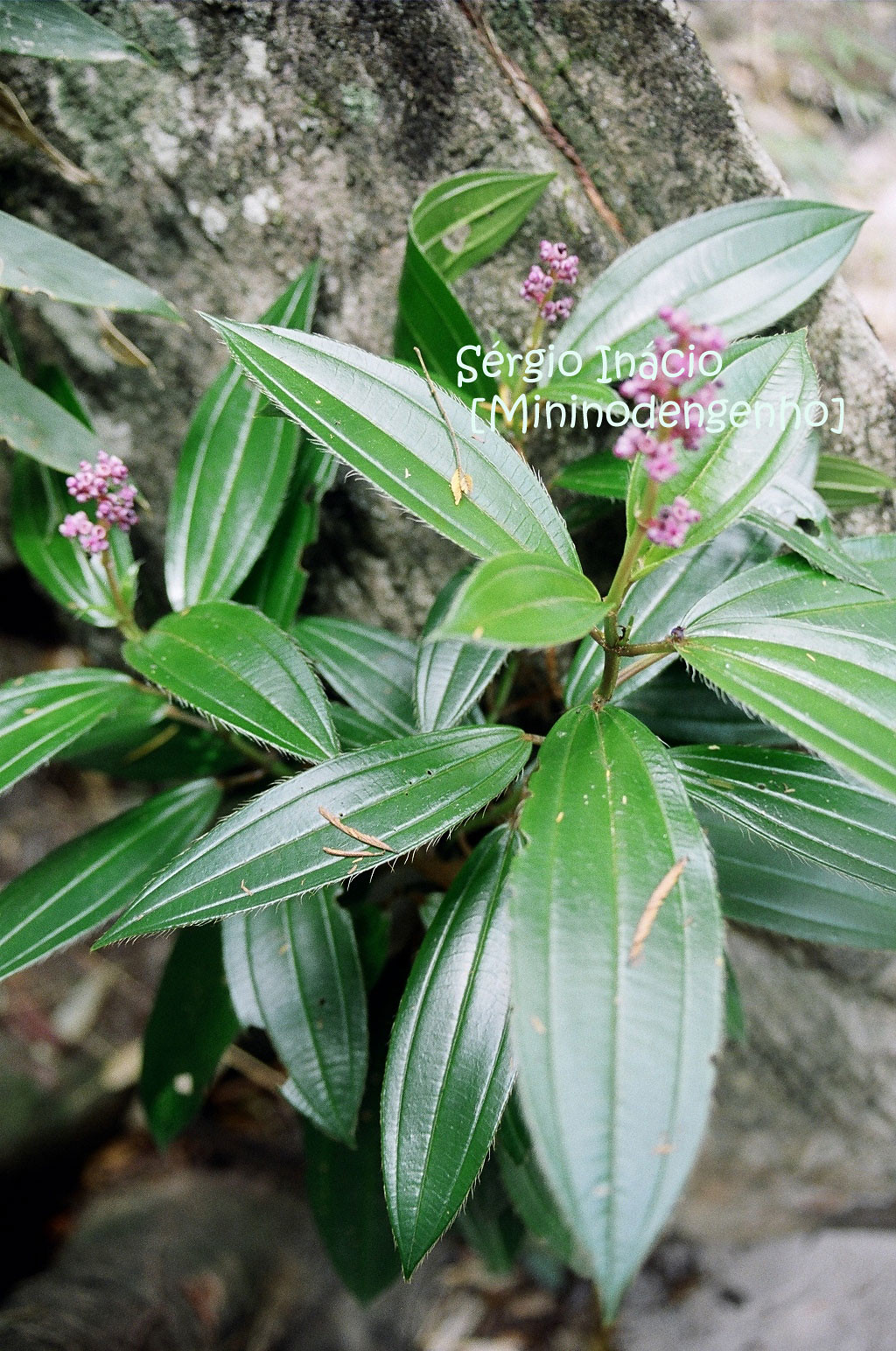The image captures a vibrant green plant with tiny purple buds clustered along the central stem, showcased in remarkable clarity. The plant stands out against a background featuring a piece of wood, providing a contrasting natural setting. The entire image is in full color, with a palette that includes shades of green, purple, and gray. No other objects, people, or vehicles are present in the photograph. White text overlays the image with the words "Sergio Inacio" at the top and "Menino Dengano" below. The scene is brightly lit by natural daylight, emphasizing the plant's details and the wooden backdrop. This well-focused, high-quality outdoor photograph draws attention to the plant's delicate features and the serene simplicity of its surroundings.